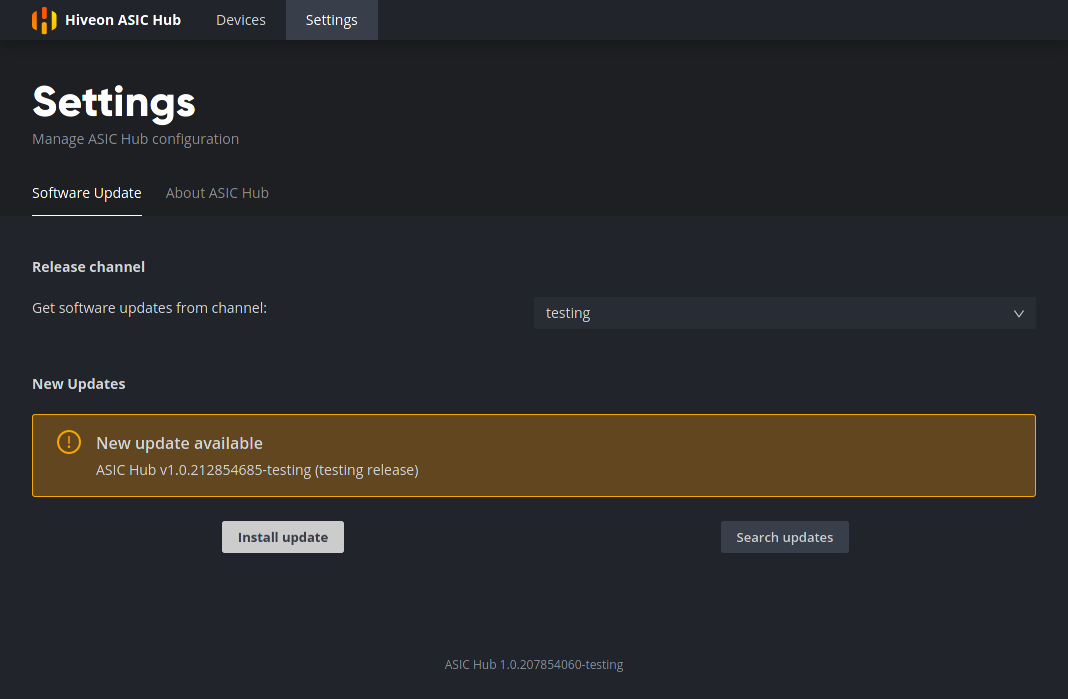Detailed Caption: 

This image showcases the update interface of the Hyvian ASIC Hub software. The interface features a sleek black background with white text for high contrast and readability. At the top, the "Devices" and "Settings" tabs are displayed, with the "Settings" tab currently selected. The section prominently displays the heading "Manage ASIC Hub Configuration," under which several options are listed.

The "Software Update" option is highlighted, allowing users to receive software updates from the "Channel Testing" release channel. Next to this is a context menu with an adjacent option labeled "About ASIC Hub."

In the bottom portion of the interface, there is a noticeable orange warning indicator. This indicator consists of an orange bar with an exclamation point inside an orange circle. The white text within this orange warning bar announces, "New update available: ASIC Hub version 1.0.212854685-testing," with the word "testing" in parentheses. Below this warning, there are action buttons: a white "Install Update" button on the left and a "Search Updates" option on the right-hand side.

Additionally, small text at the bottom of the interface indicates the current version of the software as "ASIC Hub 1.0.207854060-testing." 

Overall, this image represents an update page for the Hyvian ASIC Hub software, providing users with options to manage, understand, and update their ASIC Hub configurations.